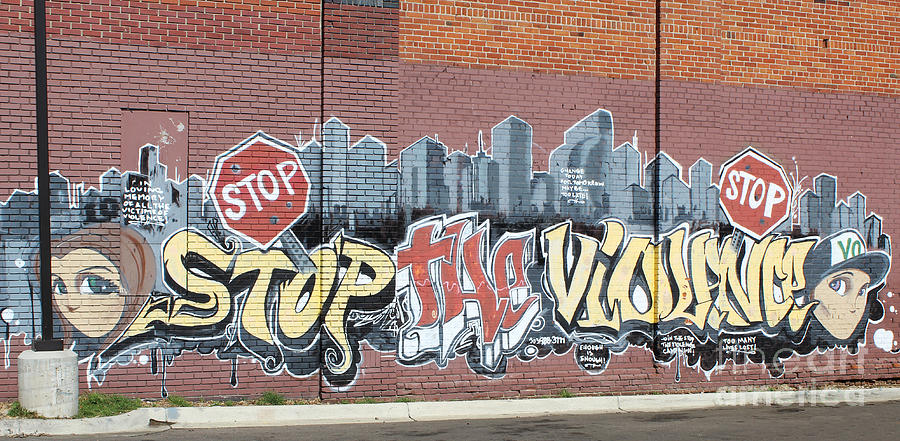The image depicts the side of a brick building, adorned with vibrant graffiti art. The brick wall, primarily reddish-brown, transitions to a lighter shade of red at the bottom, suggesting a painted lower section. Dominating the wall, the graffiti features stylized lettering that reads, "Stop the Violence," with the words 'stop' in yellow, 'the' in red, and 'violence' again in yellow. Two painted stop signs punctuate this powerful message. The artwork includes images of two faces: a man in a hat on the right and a woman on the left, both rendered in an anime style with prominent, expressive eyes but no mouths. The background is filled with a gray city skyline, replete with skyscrapers, adding depth to the mural. Additional phrases like "Too many lives lost" and "Enough is enough" are scattered across the artwork, emphasizing its call for peace. At the bottom, a hard-to-read script mentions "In loving memory of all the victims of violence." A white post or the base of a street lamp, along with sporadic grass or weeds at the curb, adds to the urban landscape. A faint watermark in the lower right corner reads "Fine Art America," hinting at the image's commercial provenance.